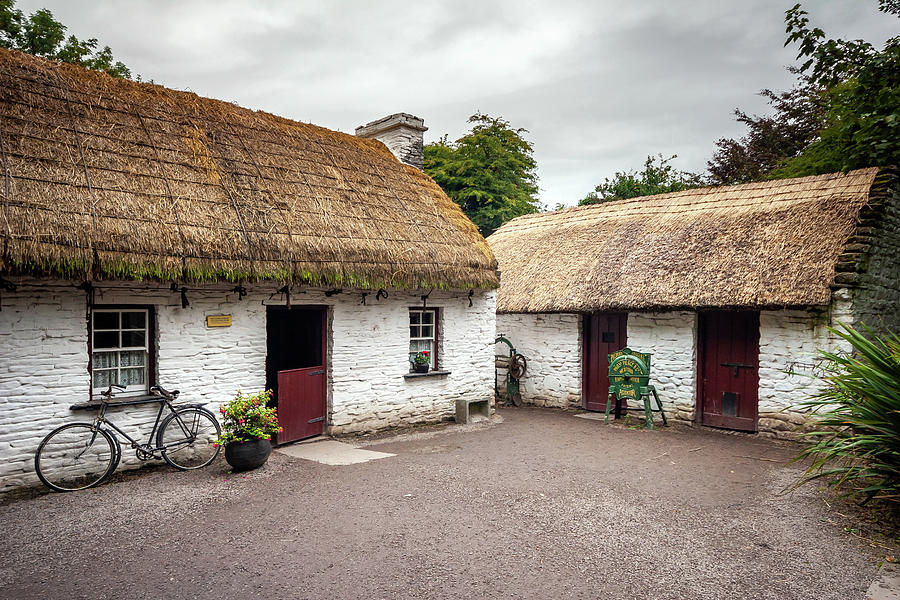This detailed photograph captures two charming white brick cottages with thatched roofs, likely situated in a European village. Each cottage features distinct characteristics and shared elements that enhance their quaint and rustic appeal. Both cottages have roofs made of tan thatched hay, giving them a traditional, rustic look, and dark brown, wooden doors.

The cottage on the left prominently displays a Dutch door, partially open, flanked by two white-framed windows. In front of the left window, a black bicycle leans against the wall, adding a touch of everyday life to the scene. On the left side of the door, a black pot holds a plant with vibrant green leaves and pink flowers. A similar green-leafed plant with red flowers graces the right window. The roof, made from neatly arranged hay, is complemented by a white brick chimney and fireplace, enhancing the cottage's cozy and inviting appearance.

The cottage on the right, also consisting of white brick, stands perpendicularly to the left cottage. It has two solid dark brown doors, between which sits a green machine with yellow text, possibly a tool or an appliance. In front of the right cottage, there is a large green bush, adding to the scene’s naturalistic charm. The ground across the scene is covered in light brown gravel, contributing to the rustic atmosphere.

An overcast sky with gray clouds looms above, adding a moody and serene tone to the image. In the background, clusters of trees and shrubs frame the cottages, completing the picturesque and idyllic rural setting.